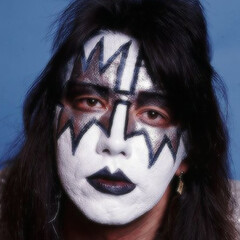The photograph depicts a close-up of a person’s face, set against a light blue wall. The individual has long, flowing black hair that cascades past their shoulders and frames their face. Their face is entirely painted white, with dramatic, black-painted lips that are pointed at the top and fade slightly toward the inner part, revealing hints of pink. Around their dark brown eyes, intricate black and gray makeup forms a pattern reminiscent of stars, extending from their forehead down to their cheeks, with three spikes at the top and bottom of the eyes and a black outline surrounding a gray or silver interior. This artwork gives an impression similar to Gene Simmons' style from the band Kiss. The person sports a tan-colored earring in their right ear, and a small section of a white shirt is visible in the corner of the image.